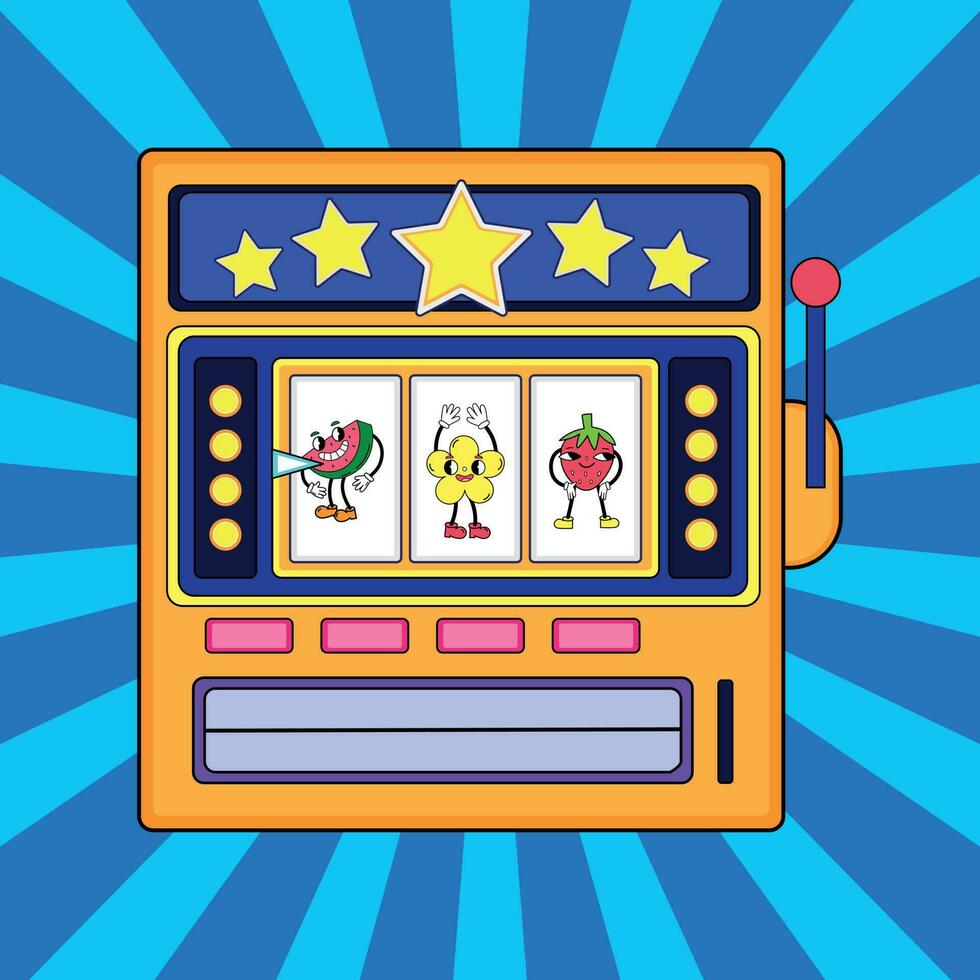This is a cartoon-style, digitally created image of a slot machine centered within a wide vertical rectangular illustration. The background features alternating diagonal stripes of light blue and dark blue, radiating outward from behind the slot machine. The slot machine itself is predominantly orange with a blue handle featuring a red dot at its end, positioned on the right side. At the top of the machine, a blue bar with a black outline displays five five-pointed golden stars, with the middle star being larger and outlined in white. Just below this bar, the dials of the machine reveal anthropomorphic characters: a smiling watermelon on the left, a smiling flower with raised hands in the center, and a strawberry with hands on its hips on the right. The slot machine's body is yellow, accented with horizontal blue stripes and yellow dots along the sides. At the very bottom, there is a gray opening, symbolizing where the money would come out. The overall scene is vibrant and playful, with a whimsical depiction of fruit characters adding to the animated charm.